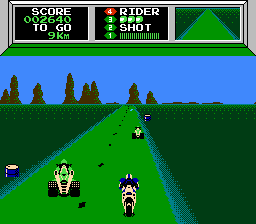This screenshot from a video game features a detailed interface and a vivid in-game environment. At the top portion of the screen, there is a prominent status bar. On the left-hand side of the bar, the text "Score: 002640" is displayed in white, with the numbers in green. Below this, the text reads "To Go: 9 kilometers" in the same color scheme – white for the text and green for the numbers.

To the right of the score, the interface shows the text "For Rider 3" followed by three green circles. Additionally, there are indicators labeled "Two Shots" and "One" with several green lines below it, suggesting some form of in-game resources or power-ups.

The main part of the screenshot shows two cars and a motorcycle driving along a green-colored road. Flanking the road is dark green grass, adding depth to the scene. The background features brownish trees set against a bright blue sky, completing the vibrant and dynamic visual depiction of the in-game world.